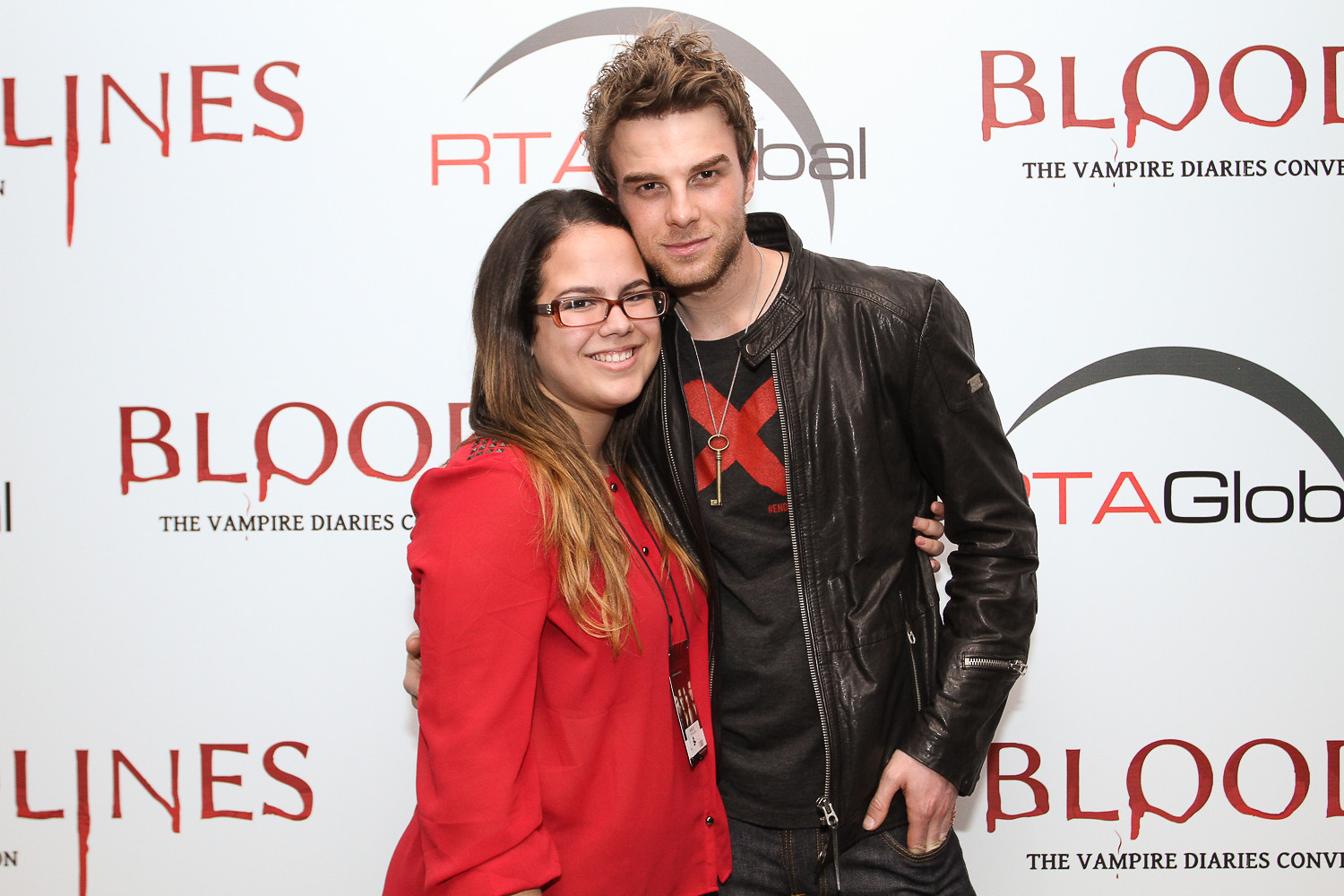This horizontally oriented photograph captures a young man and woman standing on a stage at what appears to be the "Bloodlines: The Vampire Diaries Convention," as indicated by the repeated text and graphics on the white backdrop behind them, sponsored by RTA Global. The woman, a fair-skinned young adult in her early 20s, has dirty blonde hair that falls past her shoulders and wears glasses. She is dressed in a red button-down shirt and has a lanyard around her neck, smiling warmly at the camera. Standing to her right, the man grins with a closed mouth. He has brown hair styled in a spiked or slicked-back fashion, a stubbly beard, and wears a black leather jacket over a black t-shirt featuring a red graphic, along with black jeans. He accessorizes with a key necklace. His right arm is around her back, while his left hand rests in his pocket.